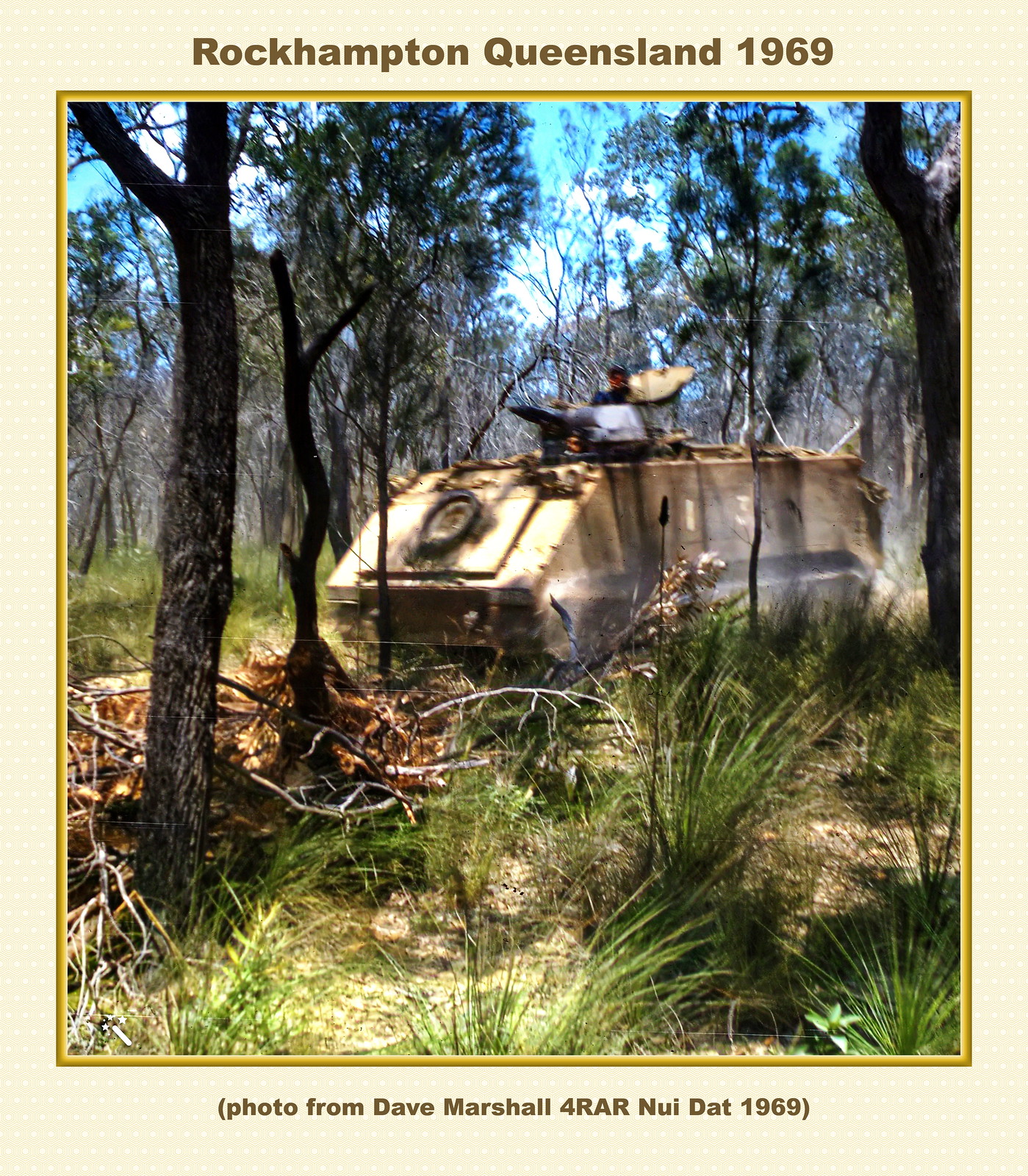This is a detailed color photograph from 1969, captured by Dave Marshall for RAR Nui Dat, with the location labeled as Rockhampton, Queensland. The image is framed with a cream-colored border and a gold line, with the text "Rockhampton, Queensland 1969" at the top and "photo from Dave Marshall for RAR Nui Dat 1969" at the bottom. It depicts a sunny day in a verdant forest with thin, green-leafed trees allowing a view of the bright blue sky with scattered clouds. In the foreground, green grass with dry patches and dead branches are visible. The centerpiece of the photograph is a heavily rusted and battered old war tank, brown in color, positioned centrally. A man stands partially out of the tank’s porthole. Although the tank’s gun is blurred, it is barely visible at the front. The overall scene appears to capture a serene yet nostalgically historical moment, reflecting the passage of time on the war relic.